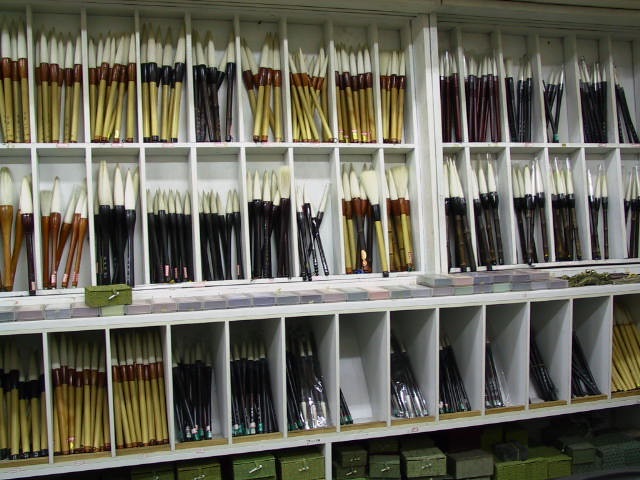This color photograph captures the interior of an art supply store, showing a detailed section of a wall filled with wooden, white compartments. Each compartment is neatly stocked with vertically arranged paintbrushes that feature uniform, precise-looking white bristles with pointed tips. The handles vary in color, with most being black or light brown, and some even show a hint of yellow and burgundy. The paintbrushes are stacked across three visible shelves, with each shelf containing 10 to 12 individual compartments. On the bottom shelf, partially visible green boxes add another layer of organization. Above the third shelf, there are mini notepads in shades of green, red, and dark purple. Some paintbrushes on the third shelf appear wrapped in plastic. The setup invites customers to walk around, select their desired brushes, and place them in one of the boxes available below the compartments. The scene is meticulously organized, reflecting the precision and variety one would expect in a well-stocked art supply store.